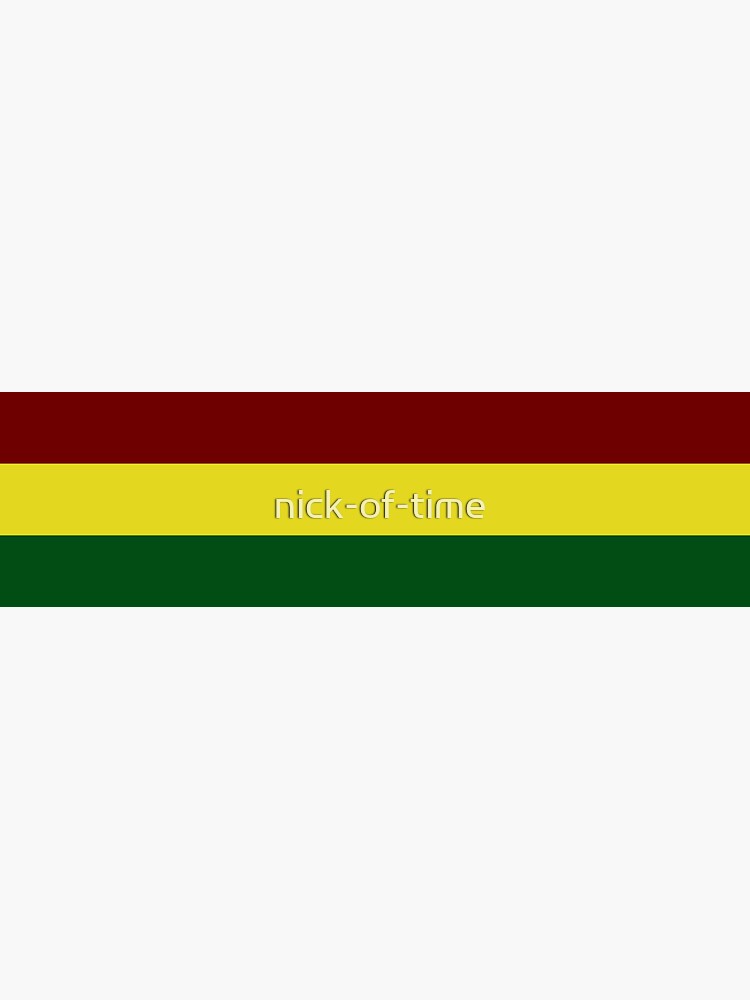The image features a flag composed of three horizontal stripes stacked vertically across the entire picture. The top stripe is a dark, burgundy red, the middle stripe is a vibrant mustard yellow, and the bottom stripe is a deep, leaf green. In the center of the yellow stripe, "nick-of-time" is written in lowercase white letters, separated by hyphens. The background of the image is predominantly white, giving it a stark, clean appearance. The flag is elongated, appearing about two to three times longer than usual proportions, and the vivid stripes and text stand out strikingly against the minimalist white background.